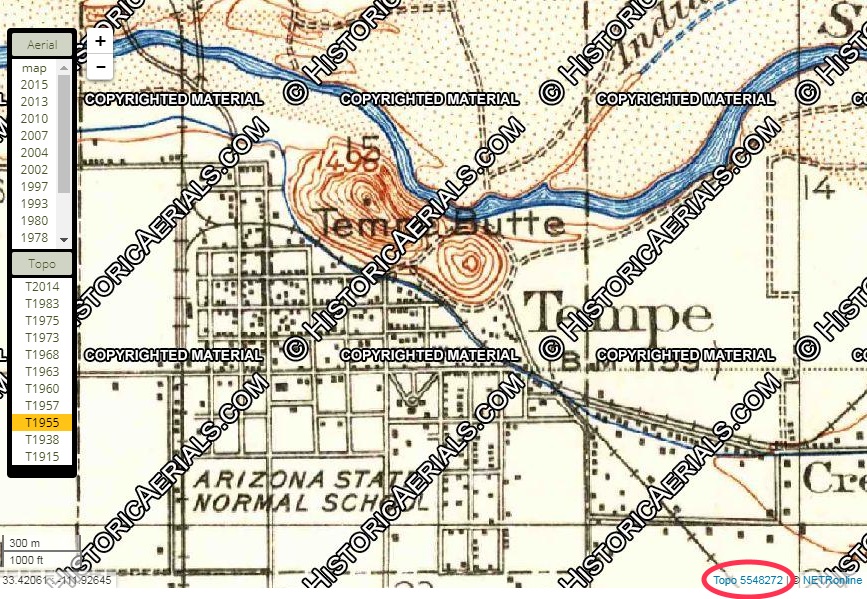This image is a scanned topographical map of Tempe, Arizona, likely hand-drawn decades ago. The map prominently features the label "Tempe" in the center and "Arizona State Normal School," indicating an early reference to Arizona State University, which is situated in this town near Phoenix. The map displays detailed geographic features, including the distinct striations of the hills and hand-drawn lakes, though it lacks specific street names. A draggable menu on the left allows viewers to select different years and styles of maps. Diagonal, repeating watermarks across the image read "historicaerials.com," indicating copyright protection. In the bottom right corner, there is a blue label that reads "Topo 5548272" circled in red. Overall, this map offers a detailed historical view of Tempe's topography.